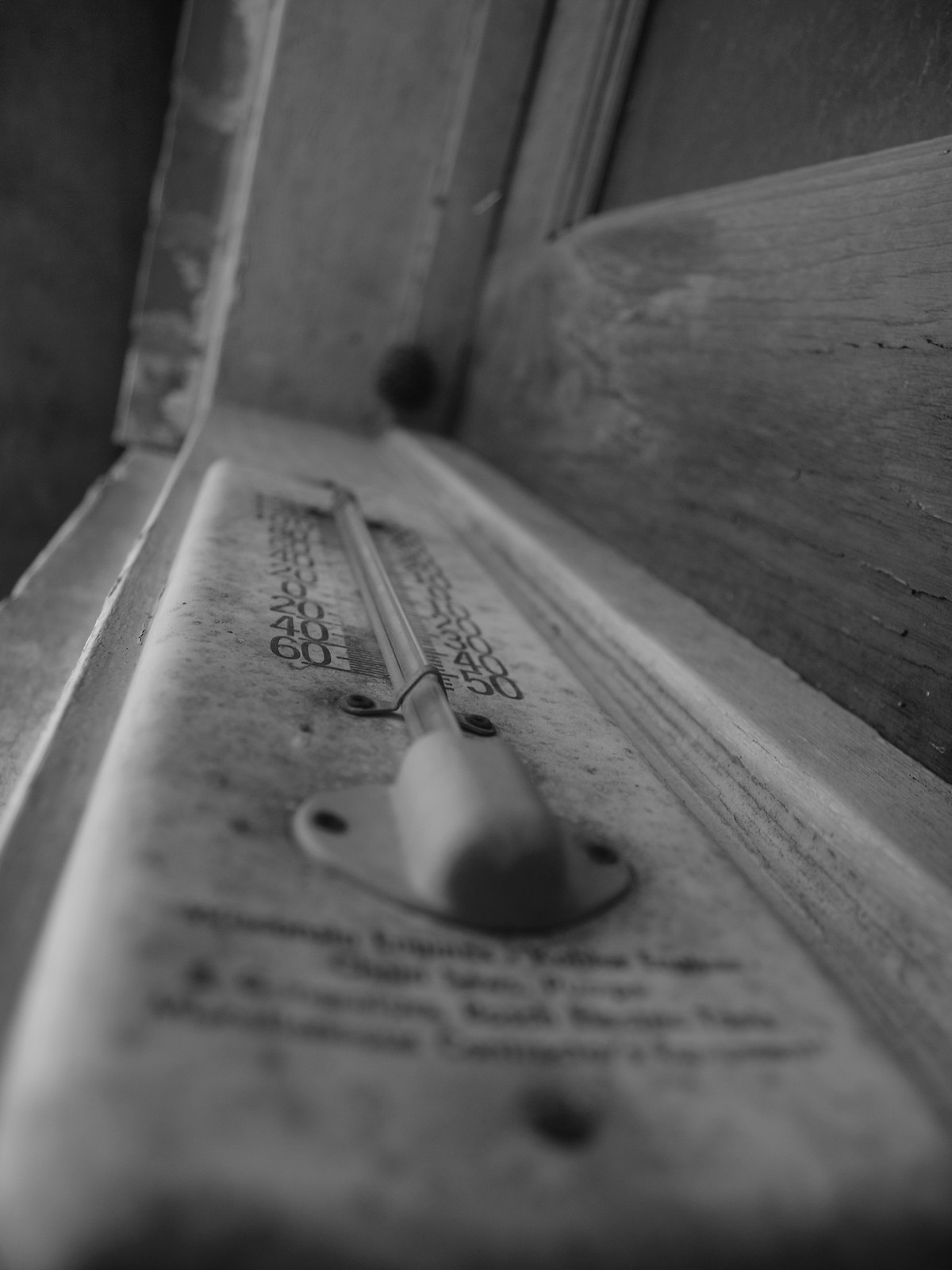This black-and-white photograph captures an old-fashioned thermometer, mounted either in a wooden window sill or door frame. The thermometer, which appears to be made of either well-worn plastic or metal, shows significant signs of age and wear. The unusual angle of the shot is taken from within the door frame or window frame, looking upwards toward the device. As a result, the top of the image features parts of the wooden frame, while the right side of the image vaguely shows what could be a window casement.

The thermometer has two columns of numbers on either side, though the exact units are unclear. These columns do not match a typical Celsius and Fahrenheit scale, adding to the antique or possibly foreign nature of the device. The thermometer is affixed with screws or nails at both the top and bottom. Though some illegible writing is present on the thermometer, its purpose or origin remains a mystery. Overall, the image presents a nostalgic glimpse into vintage temperature measurement devices and the rustic settings in which they were used.